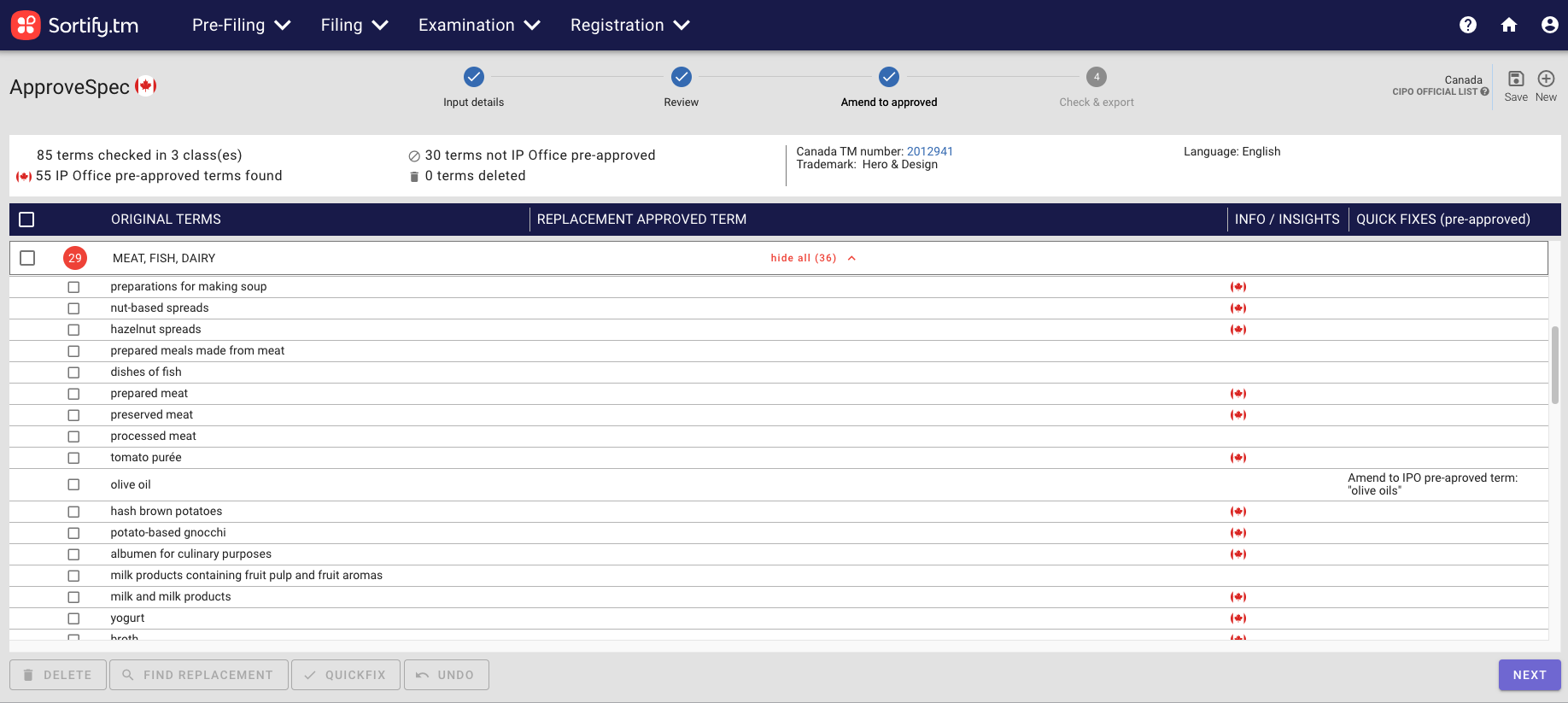The top right corner of the website features a blue background with the logo "sortify.tm" in white. Directly below, the text "Pre-Villain Examination Registration" is displayed prominently. A white circle in the upper right-hand corner contains a blue question mark icon. The central part of the page showcases a white circular icon resembling a house, suggesting it represents an image of a person or user profile.

The background transitions to gray, with the text "Approved Spec" written in black. Accompanying this is a circular icon containing the Canadian flag, followed by three circles, each with a white checkmark inside. The black text below each circle indicates the steps in the process: "Input Details," "Review," and "Amend to Approve," with the third step highlighted in bold, identifying it as the current step. A fourth gray circle marked with a white number four denotes the final step, labeled "Check and Export," indicating it hasn't been reached yet.

On the right-hand side of the page, "Canada CIPO Official List" is shown in black, alongside buttons labeled "Save" and "New." The left-hand side provides a summary: "85 terms checked in three classes," "55 IP office pre-approved terms," "30 terms not IP office pre-approved," and "0 terms deleted." Additionally, the blue text "Canada TM number 2012941" is prominently displayed, followed by "Trademark Hero and Design" and the language "English" in black text.

Towards the bottom of the page, a blue background contains white text labels for various tabs: "Original Terms," "Replacement Approved Terms," "Info/Insights," "Quick Fixes," and "Pre-Approved." Below this section, a list of items is displayed in black text, including "Meat, Fish, Dairy, Preparations for making soup, Nut-based spreads, Hazelnut spreads, Prepared meals made from meat, Dishes of fish, Prepared meat, Preserved meat, Processed meat, Tomato puree, Olive oil, Hash brown potatoes, Potato-based gnocchi, Albumin for culinary purposes, Milk products containing fruit pulp and fruit aromas, Milk and milk products, Yogurt, and Broth."

This detailed summary encapsulates the comprehensive and intricate layout of the webpage as described.